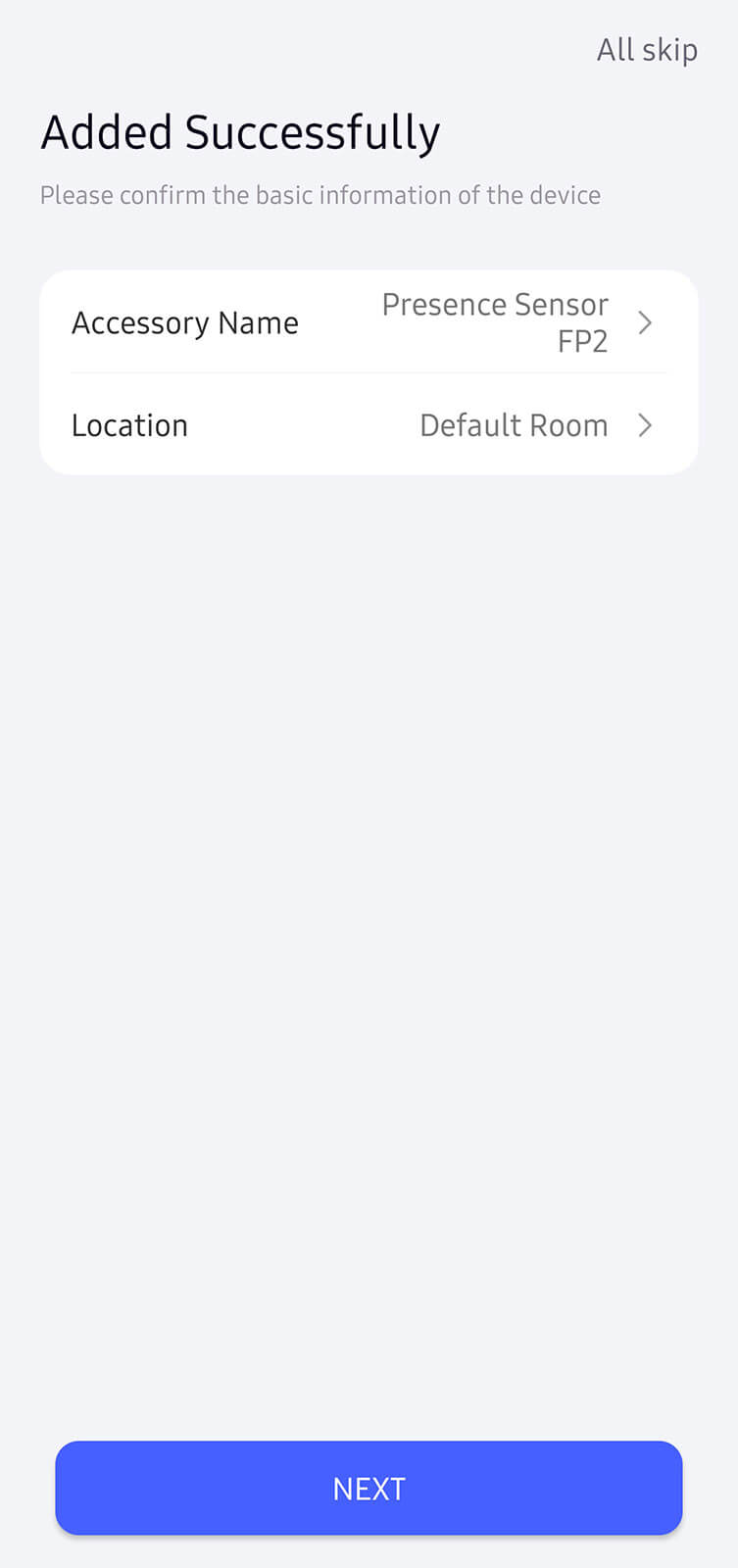The image depicts a minimalist user interface screen with a white background and black and blue text. At the very top, a confirmation message reads "Added successfully." Below this, there is a section for basic information about a device. The first item is labeled "Accessory Name," identified as "Present Sensor FP2." The second item is "Location," set to "Default Room." In the top-right corner, a small text caption says "All skip." At the bottom of the screen, there is a blue button labeled "Next." Apart from these elements, the rest of the image features empty, white spaces, emphasizing the simplicity and cleanliness of the design. No additional details or graphics are present.